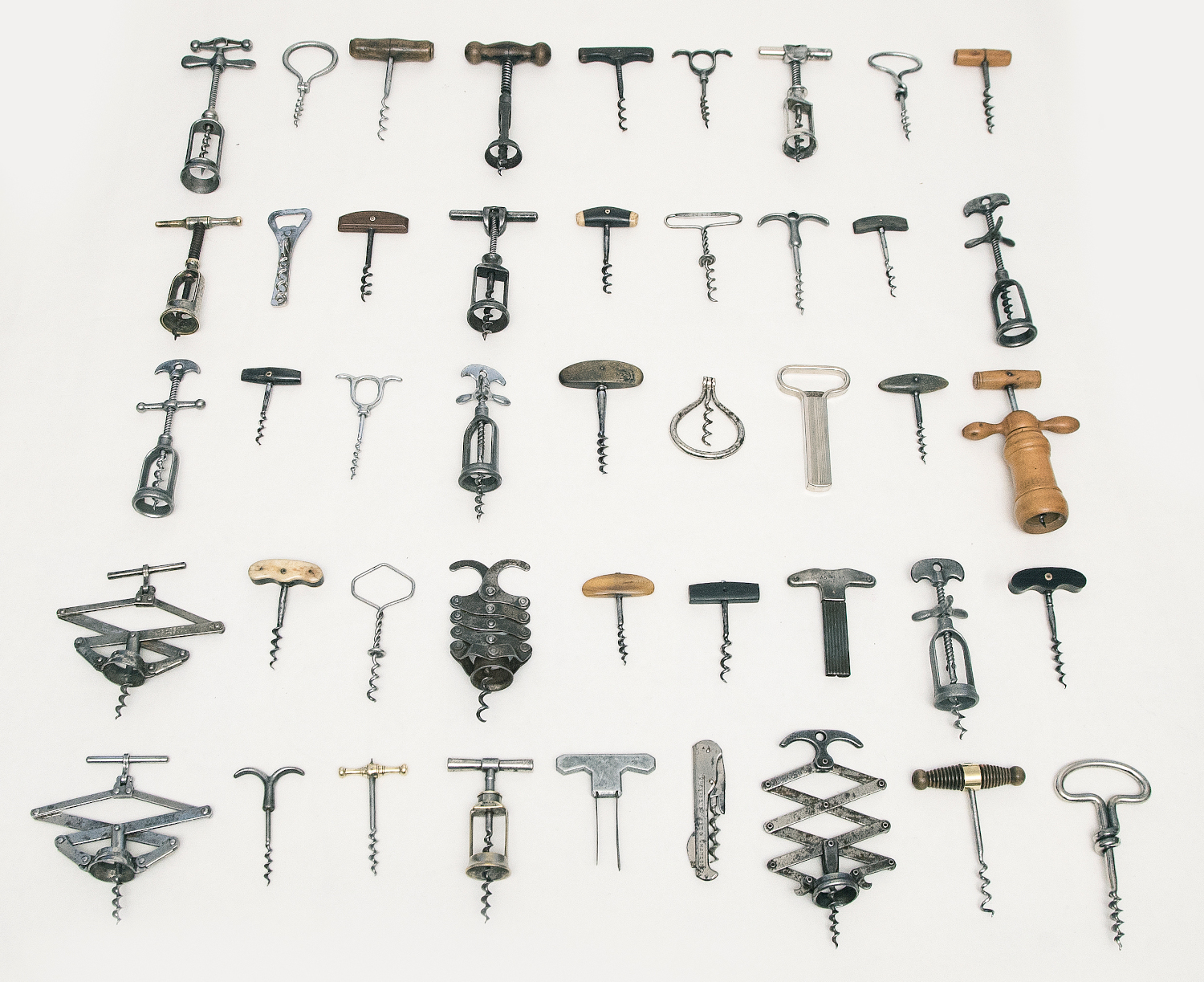This detailed photograph showcases a meticulously arranged collection of diverse corkscrews, each varying in style, mechanism, and historical period. Set against a flat surface, the collection is organized into a grid of five rows and nine columns, totaling 45 corkscrews. The colors predominantly include silver, brown, black, white, gray, and occasional rust tones, indicating different materials and levels of tarnish. The corkscrews are positioned uniformly facing downwards, emphasizing the assortment's range from antique to modern designs. Notable features include corkscrews with intricate extension arms, manually operated handles, and multi-piece mechanisms designed for effective wine cork removal. This well-composed image appears like a stock photo, likely highlighting a collector's varied and historical assortment of corkscrew devices.